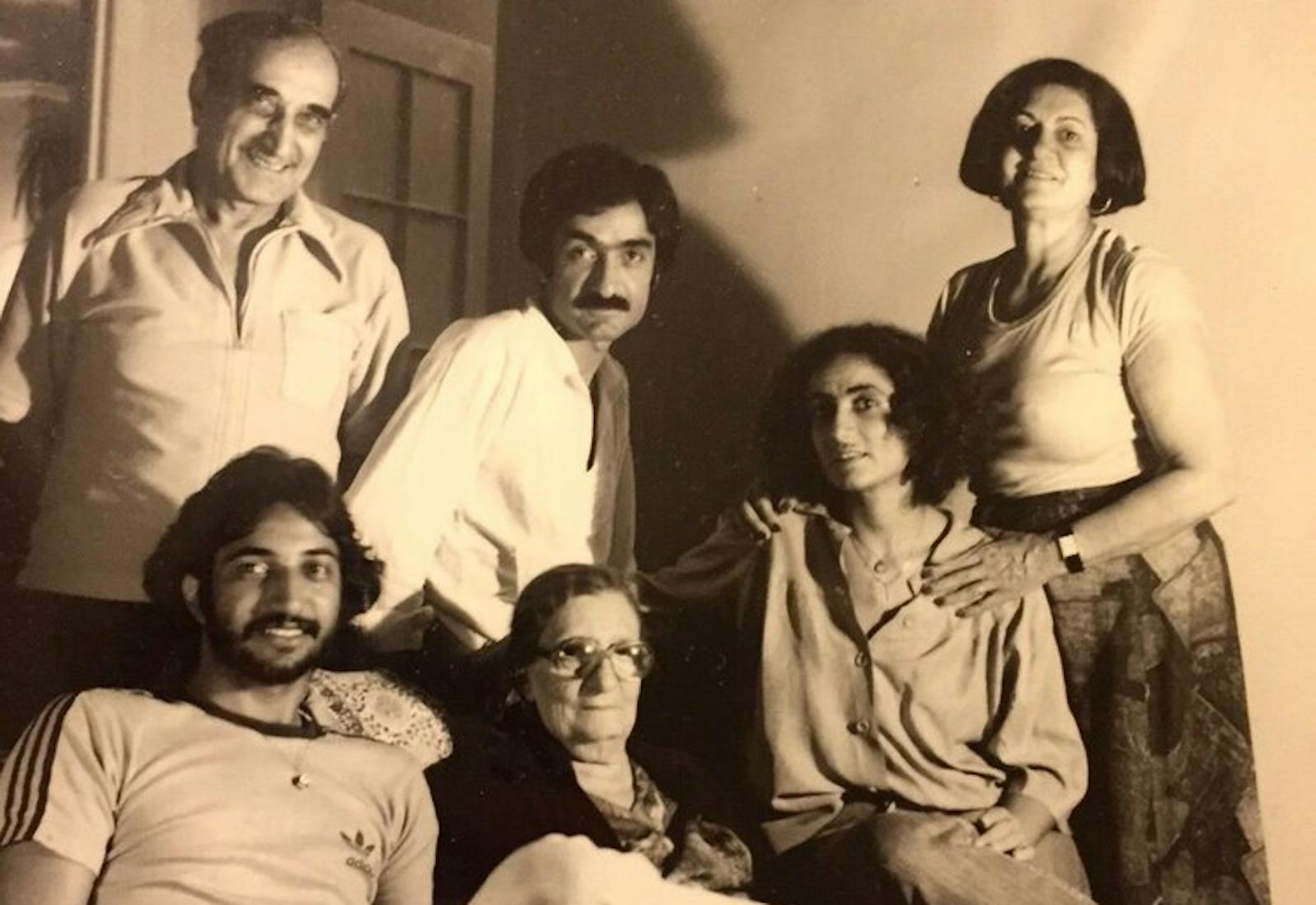This black-and-white, slightly sepia-toned photograph captures an intimate family moment inside a house, giving it a vintage feel. The image prominently features six people, with three seated in the foreground on a couch and three standing behind them. Centrally positioned, an elderly woman, likely the grandmother, is seated with thick glasses, exuding a sense of wisdom and calm despite not smiling directly at the camera. To her left is a young man with black hair, a mustache, and beard, donning an Adidas t-shirt, while to her right sits a young woman with black hair, wearing a blouse and jeans, her demeanor more reflective. 

Standing behind the seated group, the central figure is a middle-aged man with a mustache, possibly the father, flanked by another man to his right and a middle-aged woman to his left. The man on the far left is older, smiling warmly into the camera, similar to the younger men in the photo, suggesting a generational resemblance. The woman on the far right is wearing a wrist device with a black band and white body, as well as earrings on both ears, and gently places her left hand on the shoulder of the young woman seated before her. Most family members are smiling, their expressions capturing a blend of warmth and connection, further highlighting their shared heritage, likely Indian, Middle Eastern, or Persian. Shadows cast on the background wall add depth to this heartfelt family portrait.